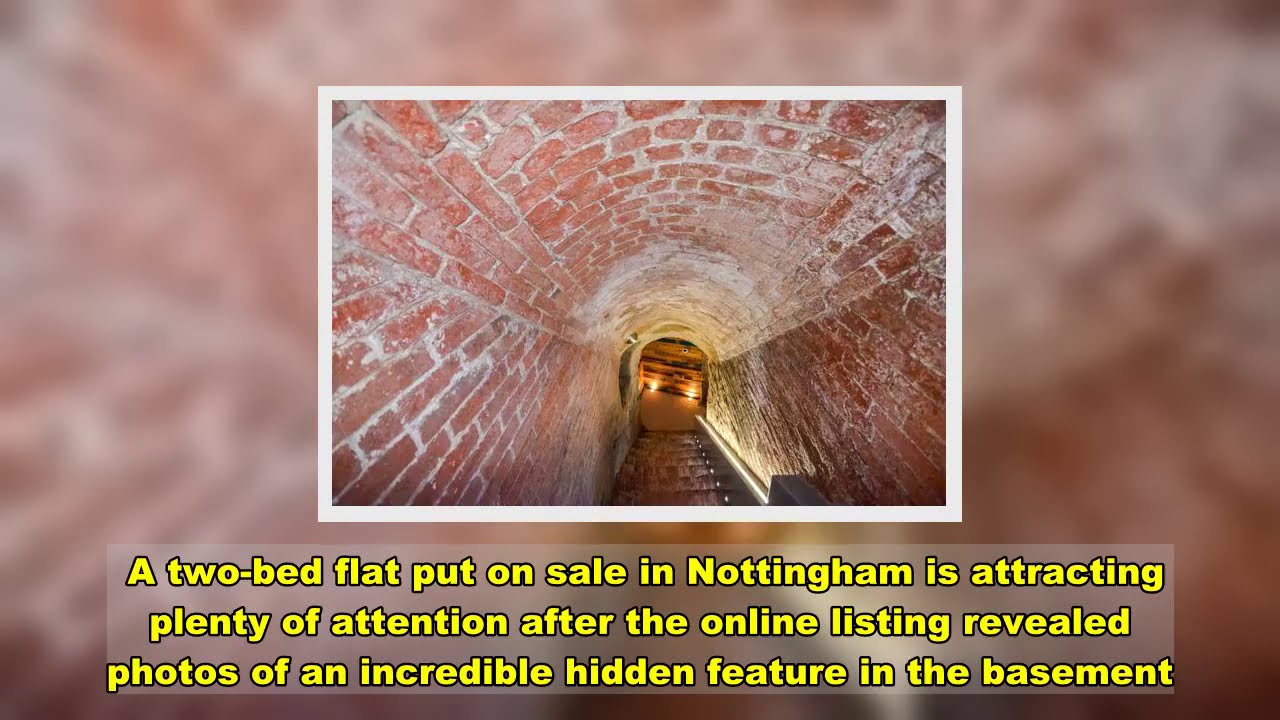The image features a centrally placed photograph of a brick-walled and brick-ceilinged stairwell leading down to a basement. The perspective is from the top of the stairs, looking downward. The bricks appear in a reddish or bright brown hue due to the lighting. Faint orange and yellow lights illuminate the bottom of the steps, partially revealing what might be a shelf or closet space, though the details remain unclear. This photograph is enclosed by a thin white border. The surrounding background is a blurred, enlarged version of the same brick stairwell image, creating an immersive effect. Beneath the photo, in bold yellow sans-serif font with a black outline, the text reads: "A two-bed flat put on sale in Nottingham is attracting plenty of attention after the online listing revealed photos of an incredible hidden feature in the basement." The text is set against a rectangle of opaque white, slightly blending into the blurred background.